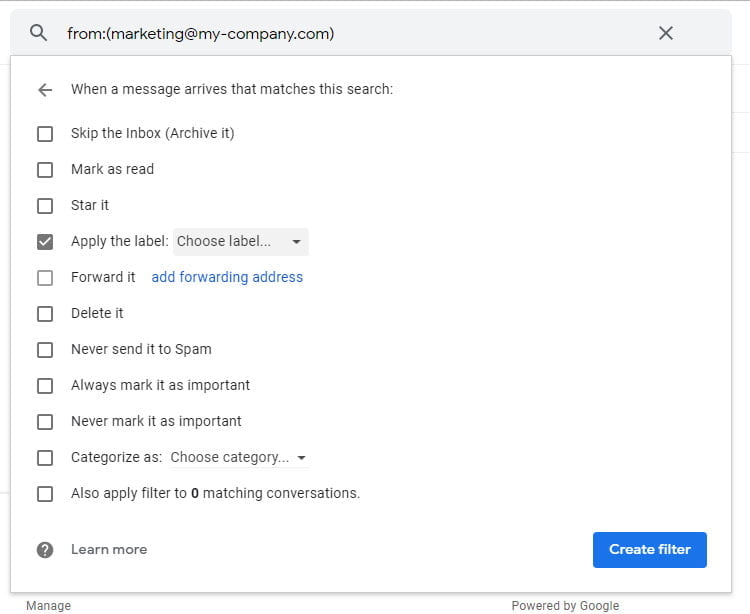The image showcases an email filter settings interface. At the top, a thin black line runs across the screen. The background of this section is gray. On the left-hand side, a dark gray magnifying glass icon is visible. Adjacent to it, in black text, it says "From..." and in parentheses, "marketing@my-company.com." To the right of this text, there is an 'X' icon. 

Below this, the background transitions from gray to white. Text in black reads, "When a message arrives that matches this search...," with an arrow pointing to the left.

A series of checkboxes are listed vertically on the left-hand side, allowing users to customize their email filtering preferences. These checkboxes have black outlines and white interiors, except for one that is checked. When a box is checked, the interior turns gray with a white checkmark.

The first option reads, "Skip the Inbox (Archive it)." The second option is "Mark as read." The third says "Star it." Following this, the fourth option, which is checked, reads, "Apply the label:" with a gray rectangle to the right that says "Choose label..." accompanied by a downward-pointing black arrow.

The additional options include:
- "Forward it" with a blue link next to it that says "Add a forwarding address"
- "Delete it"
- "Never send it to Spam"
- "Always mark it as important"
- "Never mark it as important"
- "Categorize as: Choose category"

At the bottom of the list, it reads, "Apply filter to matching conversations," with the number of matching conversations specified. Finally, in gray text at the very bottom, there is a link that says "Learn more."